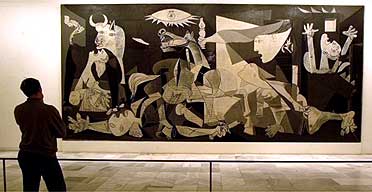In this detailed photograph taken inside a museum, a man is seen standing behind a black steel guardrail, engrossed in observing Pablo Picasso’s renowned painting, "Guernica." The man's silhouette, positioned on the left side of the image, shows him with his chin resting on his hand and head slightly cocked to the left, suggesting deep contemplation. Wearing long pants, a sweater, and sporting short hair, he stands on a tiled floor under soft lighting, which reflects off the light-colored wall.

Dominating 85% of the photo, the monumental "Guernica" is a long rectangular masterpiece occupying nearly the entire wall. The painting's dramatic dark gray and black background contrasts sharply with shades of white and various beiges. This abstract artwork is chaotic, featuring multiple disconcerting elements: a bull in the upper left, scattered human limbs, hands raised in despair, and fragmented faces. Among these elements, a sun-like eye stands out at the center left, contributing to the painting’s overwhelming sense of anguish and turmoil. The person’s contemplative stance underscores the complex, thought-provoking nature of Picasso's depiction of wartime suffering and chaos.